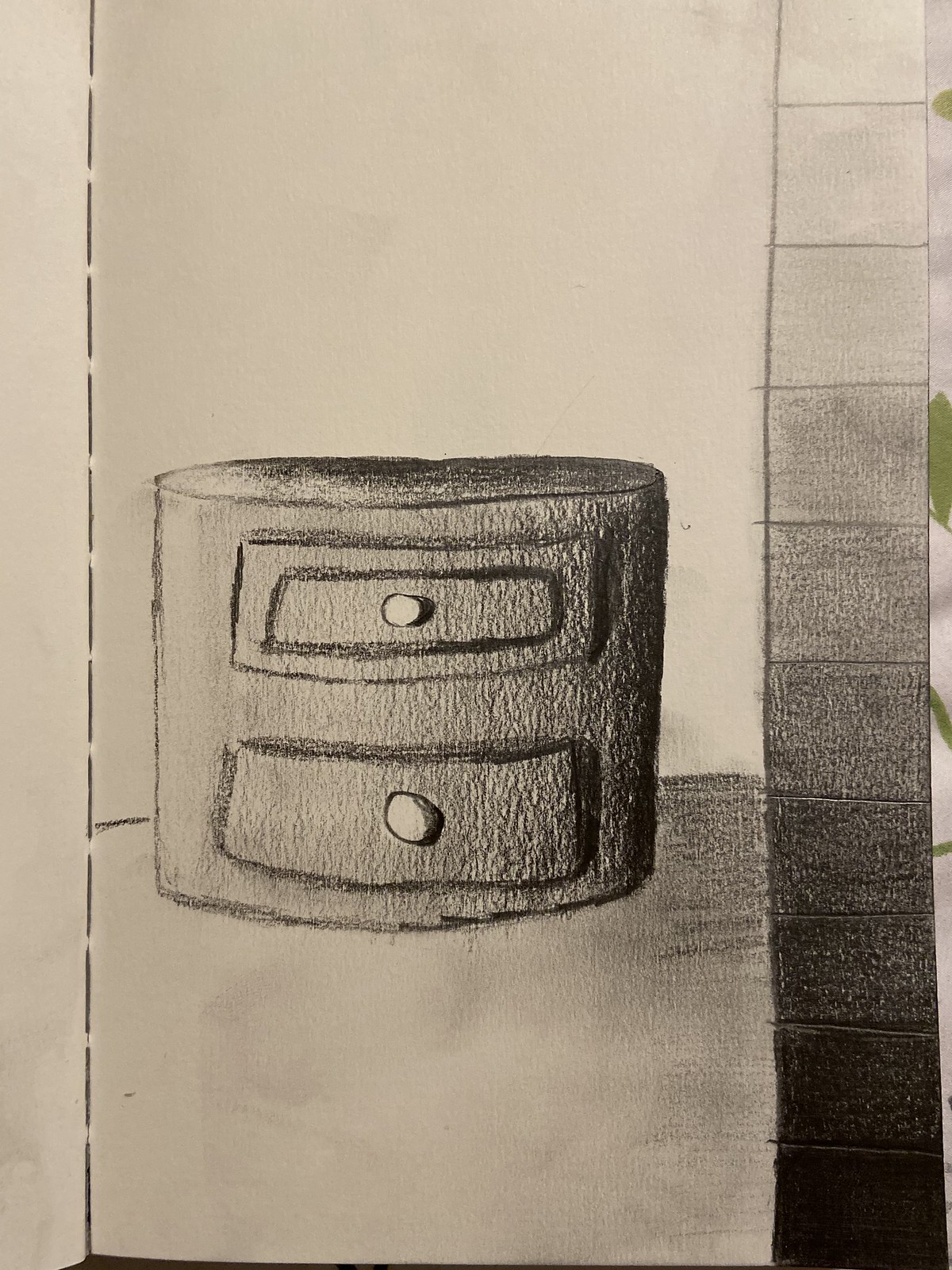The photograph captures a detailed pencil sketch on a page from a white sketchbook. Centrally positioned is a drawing of a two-drawer, oval chest of drawers, which appears to have been created using a charcoal or regular pencil. The chest's drawers are rectangular with two circular knob holes in the center. To the right of this centerpiece, extending vertically along almost the entire length of the page, is a strip divided into square segments. These segments depict a gradient color shading that transitions from white at the top to completely black at the bottom. Adjacent to the chest, someone has attempted to shade an area to represent the floor, adding a dimensional effect to the sketch. A dashed line running vertically marks the inner spline of the book. The upper left portion of the page remains predominantly white, and the overall image has a vertical rectangular shape. There are no words, text, or print visible in the photograph.